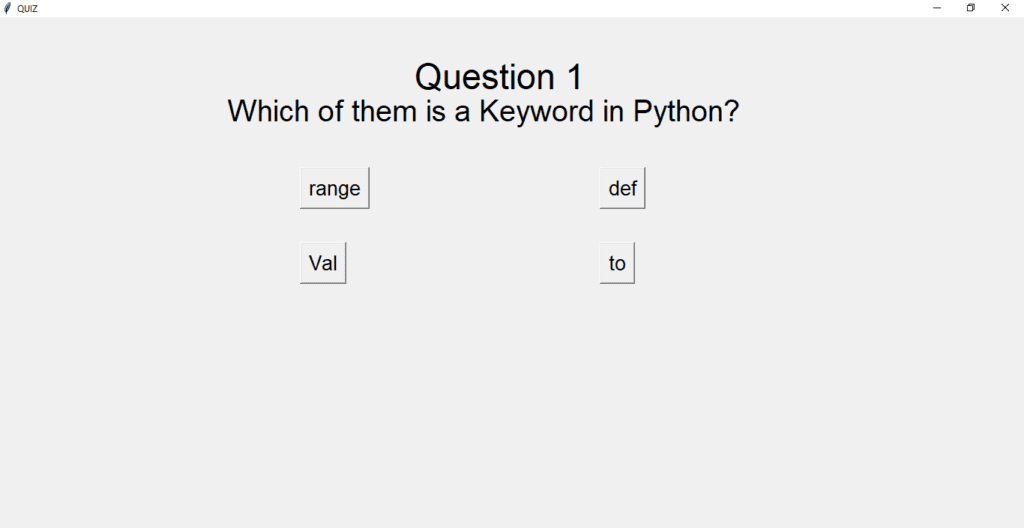The image depicts a quiz page with a minimalistic design. The background is a light gray, providing a plain canvas for the content. At the very top left corner, the word "Quiz" is visible, indicating the context of the page. Centered at the top of the page in large black font is the text "Question 1".

Directly below this heading, still centered but in a slightly smaller black font, is the question: "Which of the following is a keyword in Python?". Below this question, aligned in the middle of the page, are four options for the user to choose from, each spaced distinctly:

- "range" (typed in lowercase)
- "def" (typed in lowercase, with "d-e-f" specified in the description)
- "to" (typed in lowercase)
- "Val" (typed with an uppercase "V" and lowercase "a-l")

The options are listed in a smaller font compared to the question and are evenly spaced to maintain clarity.